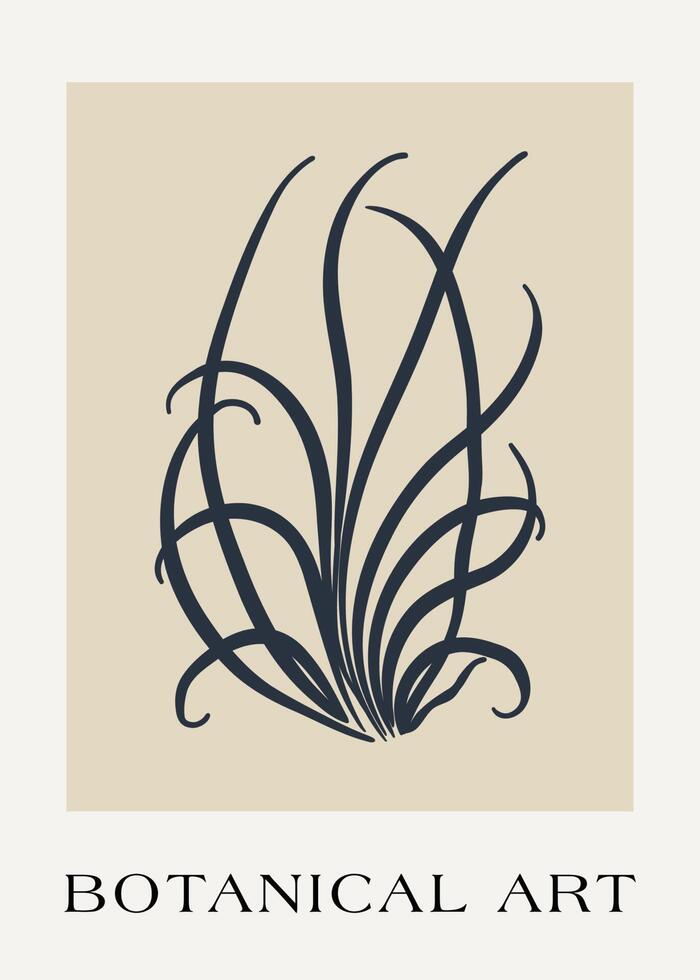The image is an artwork titled "Botanical Art," depicting a plant-like structure with multiple black stems and branches emanating from a central point on a light beige canvas. The slender branches are long and thin, devoid of leaves, giving a minimalist aesthetic. The artwork is framed by a gray border that enhances its rectangular beige background. At the bottom of the image, outside of the beige area, the phrase "Botanical Art" is inscribed in black text, emphasizing the theme of the piece. The overall presentation suggests a poster or artistic representation focused on botanical forms.